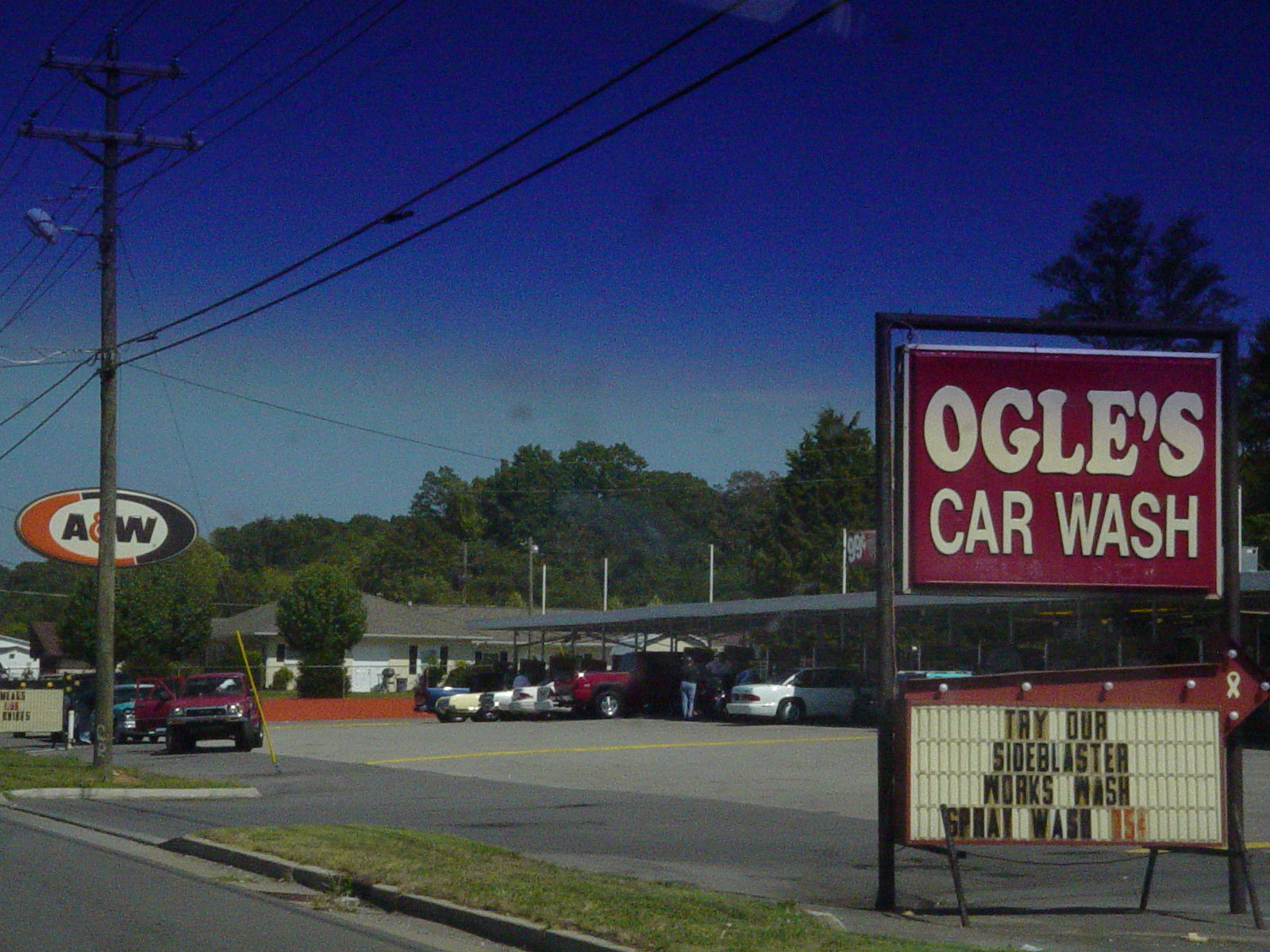This 1990s photograph captures a sunny day at Ogle's Car Wash, evidenced by the sign with a red background and white letters that reads, "Ogle's Car Wash." Below this main sign, a marquee displays, "Try Our Side Blaster Works Wash Spray Wash $0.75." The image, characterized by a low-resolution quality typical of that era, depicts numerous cars lined up in various bays under a large canopy that extends from the middle to the right side of the car wash area, viewed from the street into the parking lot.

In the bottom left-hand corner, a street runs diagonally from bottom left to the left edge of the image, bordered by curbs and patches of grass. A driveway leads into the car wash and adjacent businesses, with a utility pole and several cars parked nearby. In the left background, an A&W sign hints at a drive-thru or restaurant. The surrounding area includes green-leaved trees and what appears to be residential buildings, suggesting a mixed commercial-residential neighborhood. In addition, a family standing by one of the cars hints at the possibility of a road trip, contributing to the nostalgic tone of this photograph.